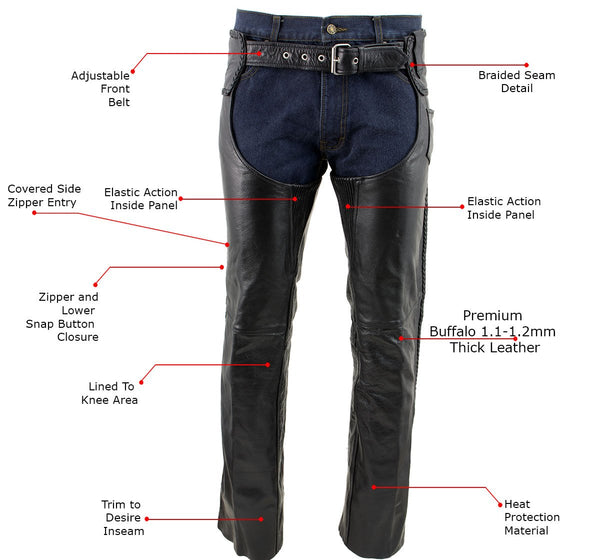The image features a detailed diagram of black leather chaps worn over dark blue denim jeans, all set against a plain white background. The chaps are secured with an adjustable front belt at the waist. Various red lines with black print are used to label specific features of the chaps: braided seam detail at the waist, elastic action inside panels at the inner thighs, and a covered side zipper entry along the thigh. Further descriptions include a premium buffalo leather thickness of 1.1-1.2 millimeters at the knee, heat protection material at the ankles, and a lined knee area. Additionally, the diagram notes a zipper and lower snap button closure and specifies that the inseam can be trimmed to desired length. These annotations offer a comprehensive guide to the chaps' construction and functional design elements.